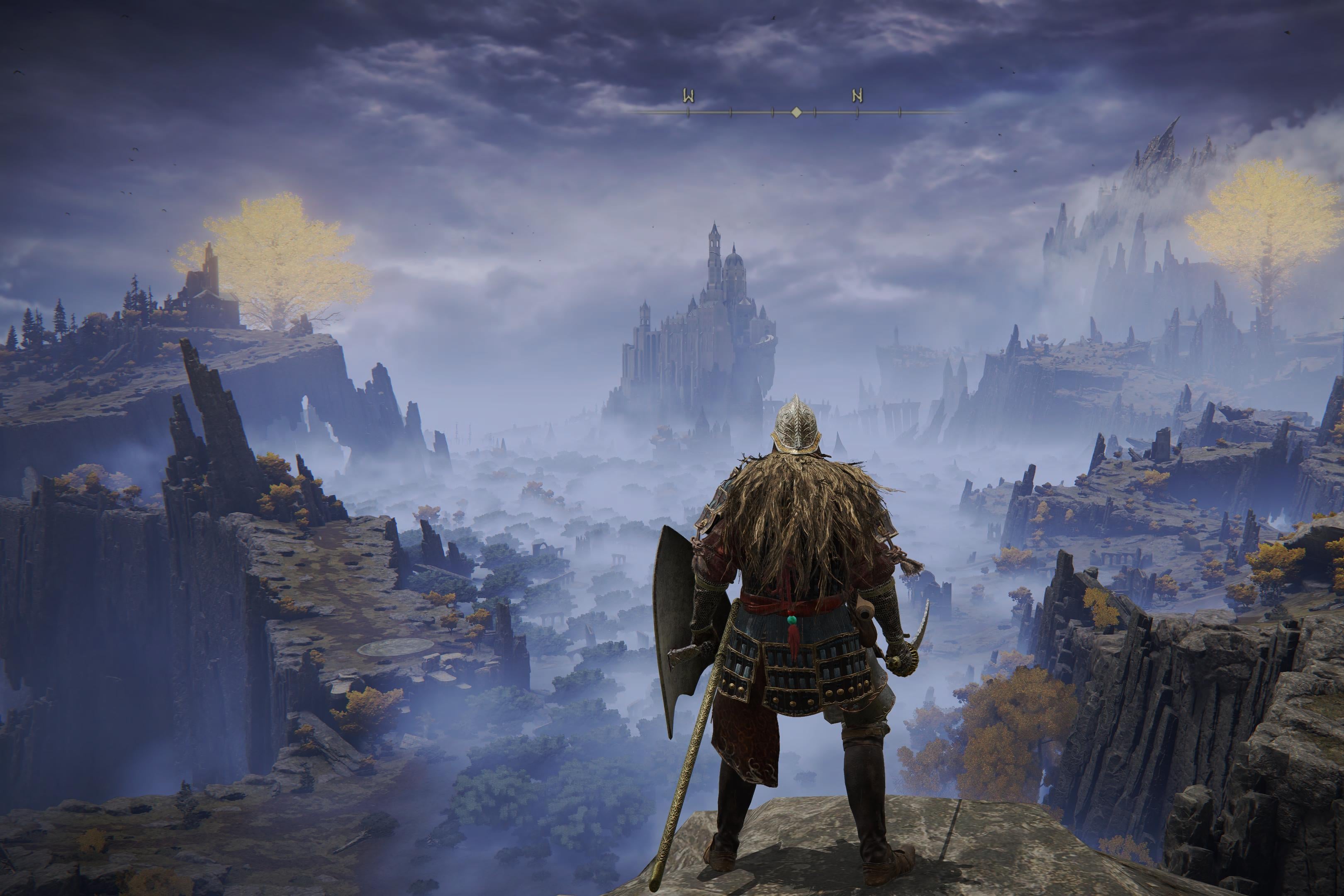This image appears to be a richly detailed, painterly concept art likely for a video game, showcasing a warrior with their back to us. The warrior is clad in dark, protective clothing reminiscent of traditional Japanese armor, characterized by slatted, plank-like elements. He dons a helmet and has mane-like, scruffy hair or a cape flowing behind him. Equipped with a shield and sword, he stands on a jagged clifftop, gazing over a vast, rugged landscape dotted with additional cliff faces and mountains. The scene is brooding with a dark, cloudy sky, hinting at an imminent storm. Central to his view is a distant castle emerging from a rocky outcrop, suggesting it as his likely destination. Off to the left, a smaller house or structure can be seen among the wilderness, enhancing the expansive and foreboding atmosphere of the scene.